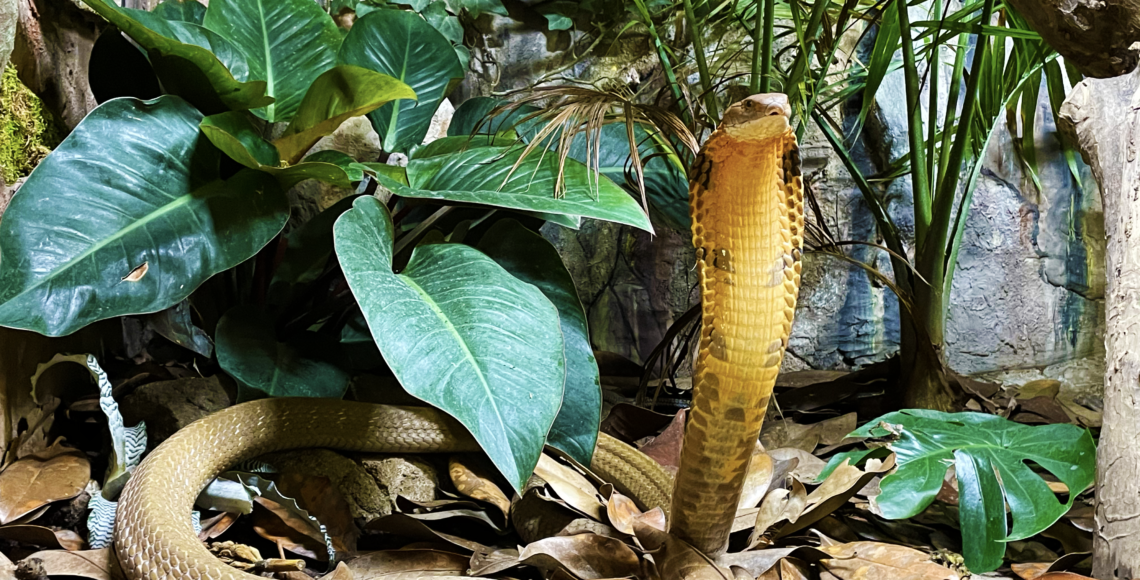This rectangular, horizontally oriented photograph vividly depicts a captivating scene with a prominent snake, likely a cobra, as its focal point. The snake is standing erect, with about the top third of its body, including its head, raised about two feet high. Its hood is flared out, revealing a yellowish belly, while the top of its head and its neck exhibit a darker, greenish-brown or mottled copper hue. The snake's body gradually darkens as you move downward, transitioning to almost completely dark scales. The lower part of its body lies coiled on the ground, trailing behind the raised portion, curling off to the left before looping forward towards the foreground and disappearing out of the bottom of the image.

The environment appears somewhat artificial, suggesting the snake might be inside a cage. To the left of the snake stands a large green plant with broad leaves, while another fern-like, spiky plant is situated behind it to the right. The snake rests on a ground covered with fallen, brown leaves, adding a naturalistic touch to the scene. A prominent gray rock or rocky area is visible in the background, reinforcing the setting as a carefully constructed habitat. The overall composition of the photograph suggests a deliberate arrangement to highlight the striking presence of the cobra amidst its surroundings.